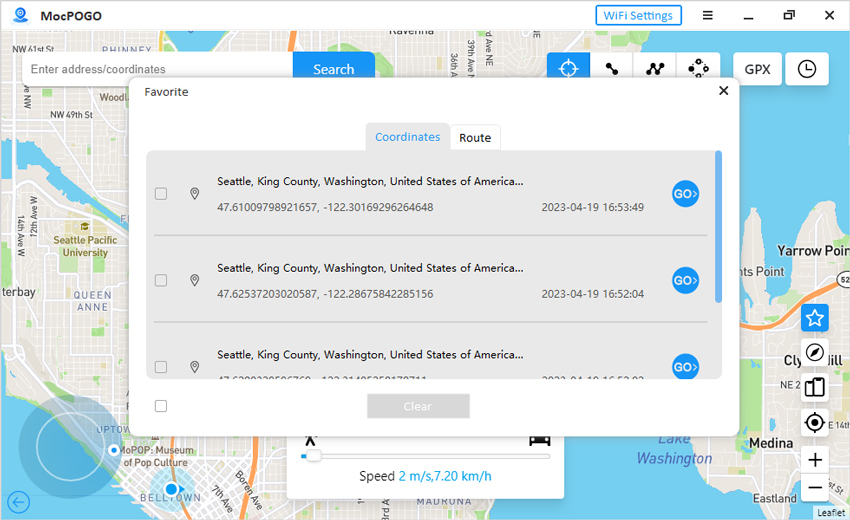This is a detailed screenshot of a map application or website displayed on a computer screen. The interface features a white banner running horizontally across the top, slightly wider and taller than usual. On the upper left of the banner, it reads "POGO M-O-C" in uppercase letters, with a small camera icon positioned to the left of the text. To the right edge of the banner, various icons are visible, including Wi-Fi settings, a blue rectangular outline, and standard browser icons.

Below the banner, a map background dominates the screen. In the upper left of this map area, there's a white input box for entering an email address, accompanied by a blue search button. To the right of this search box, a selection of icons is available, presumably for different functionalities within the map application.

Centrally superimposed on the map is a large rectangular box. The upper left corner of this box reads "Favorites." Inside the box, there are two labeled tabs: "Coordinates" and "Route." The "Coordinates" tab is selected and highlighted in gray. Beneath these tabs, three different addresses in Seattle, Washington are displayed, each accompanied by corresponding coordinates, a date to the right, and a blue "Go" button at the end. Each address also has an associated checkbox to its left. At the bottom of this rectangular box, a "Clear" button is present, though it is grayed out, indicating it is inactive until an address is selected for clearing.